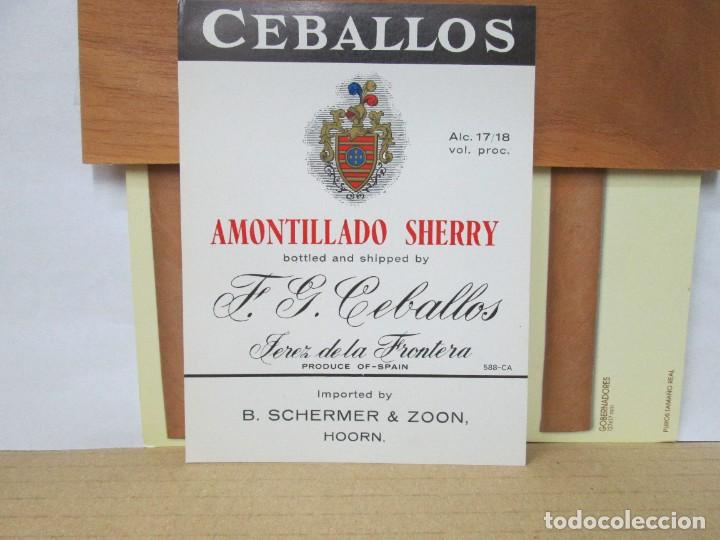This image features a promotional poster for Amontillado Sherry, measuring approximately two feet tall and two feet wide. At the top of the poster, the name "CEBALLOS" is prominently displayed in white capital letters against a black rectangular background. Below this, there's an intricate family crest adorned in red, blue, and gold. Beneath the crest, in bold red capital letters, the words "Amontillado Sherry" are inscribed, followed by the details "modeled and shipped by F.G. Ceballos" written in cursive. Further down, the text "Ferreira de la Frontera" appears, also in cursive. The bottom section of the poster, printed in plain black lettering, states "Produce of Spain, imported by B. Shermer and Zun, H.O.R.N." In the bottom right corner of the image, the brand name "Todo Coleccion" is repeated twice in white letters. The poster is shown leaning against a wooden wall and is positioned on top of a wooden table.